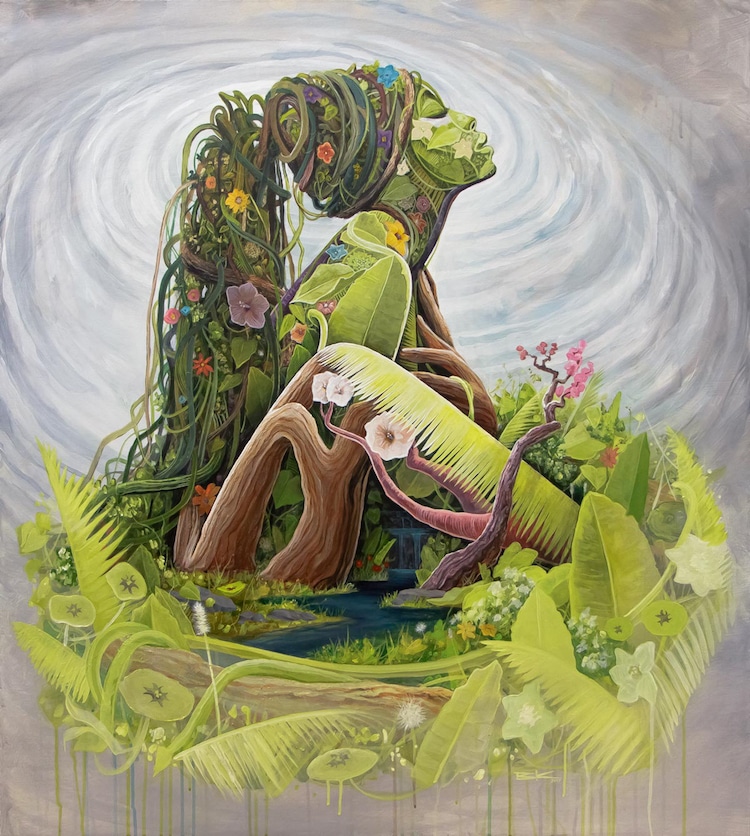This digital artwork, possibly resembling a painting, features a striking, abstract representation of a woman symbolizing Mother Nature. The central focus is on a circular, bird's nest-like structure at the bottom, composed of various shades of brown interspersed with lime green leaves and mushroom-like forms. A blue stream with a waterfall cuts through the middle, enhancing the mystical feel of the image.

Above the waterfall, a woman is depicted in profile, facing the upper right. Her form is intricately made of branches, stems, leaves, and flowers. Her hair cascades like a long ponytail composed of vines, now transformed into a vibrant mosaic of botanical elements. Her shoulder area is crafted from green leaves and colorful blooms, while her chest and hand resemble tree trunks and branches. The background swirls with hues of white and blue, adding to the ethereal quality. 

The base of the image is adorned with dripping paint, streaking in greens and blues, contributing to the overall fluidity and organic essence. This highly detailed and imaginative piece evokes themes of nature, creation, and earth's intrinsic beauty.